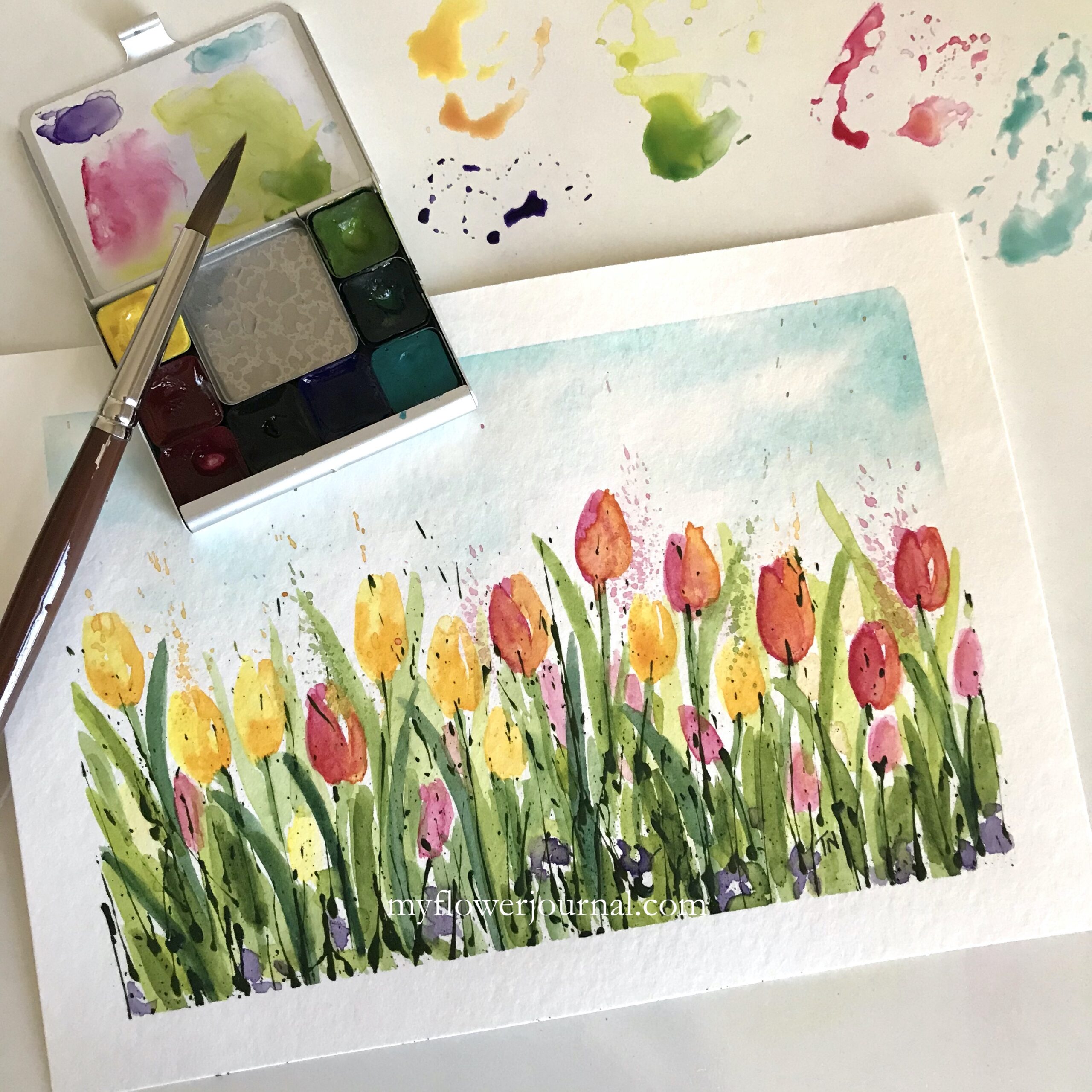The photograph showcases a vibrant watercolor painting of tulips set against a clear blue sky dotted with white clouds. The tulip blooms in shades of yellow, red, pink, and purple are accented by green stems and leaves, all beautifully depicted at the bottom of a white paper. The painting is accompanied by a watermark, "myflowerjournal.com," suggesting it's part of an advertisement or a creative journal. Surrounding the art, blobs of watercolor paint in hues of orange, yellow, green, pinkish-red, and blue decorate the white background. Positioned above the painting is a compact metal watercolor kit, with compartments of green, blue, red, and yellow paint, and across it rests a paintbrush with a brown handle and silver tip. Additional watercolor mixes, a goldenrod yellow, deep violet, light green, orangey-red, and teal, further highlight the artistic setting, enhancing the painterly atmosphere captured in the photo.